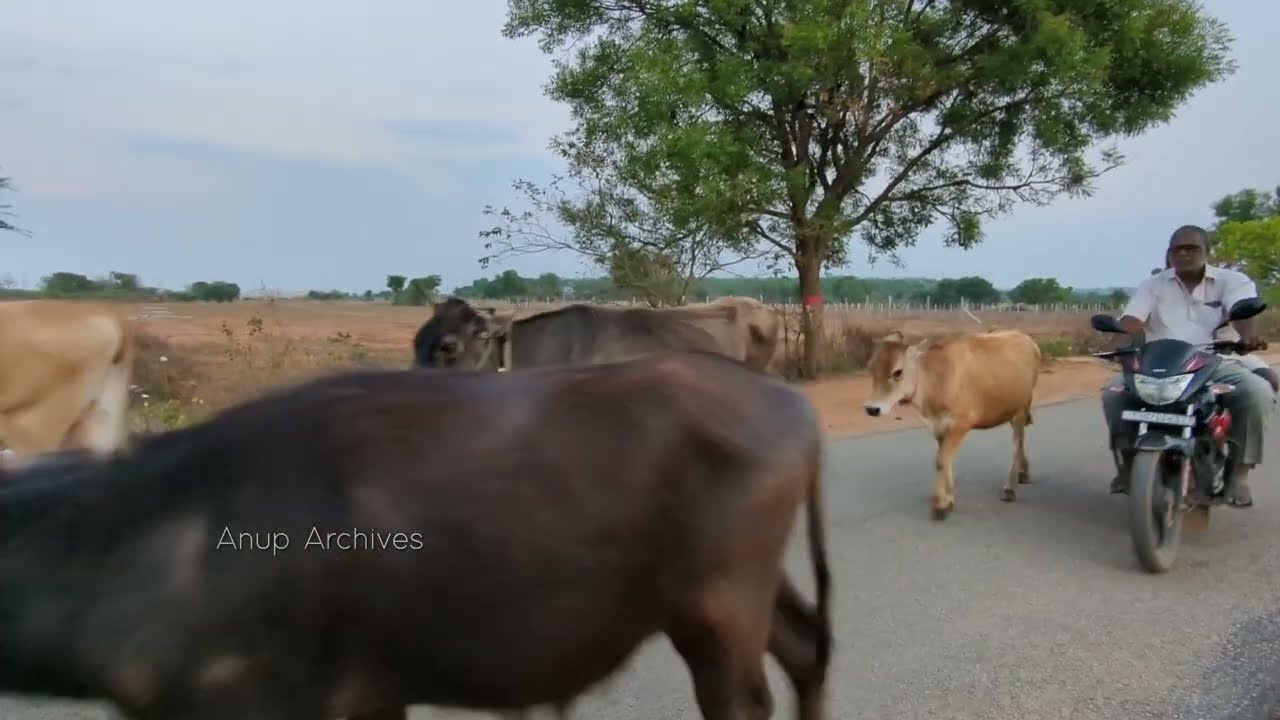In this rural outdoor scene, a dirt road sweeps from the middle right down to the lower left of the image. Riding towards us on the right side of the road is an African-American man on a motorcycle, wearing sunglasses, a white shirt, and green or yellow pants. There might be a second person seated behind him. 

To his left, a light brown cow keeps pace, while in the bottom left corner of the image, a darker brown cow faces and moves leftward. Above this cow, slightly behind and to the right, another dark brown cow follows the flow. Further up on the left, partially off the image, the back of yet another light brown cow is visible, continuing the procession off the frame.

In the mid-background, a lone tree stands adjacent to the road, its green leaves providing contrast to the surrounding field, which is filled with light brown, dying foliage. The horizon is dotted with a grove of trees, and the sky above is a light blue, indicating daylight. There are various bushes scattered around, with dirt patches visible, adding to the rustic charm of this pastoral scene.